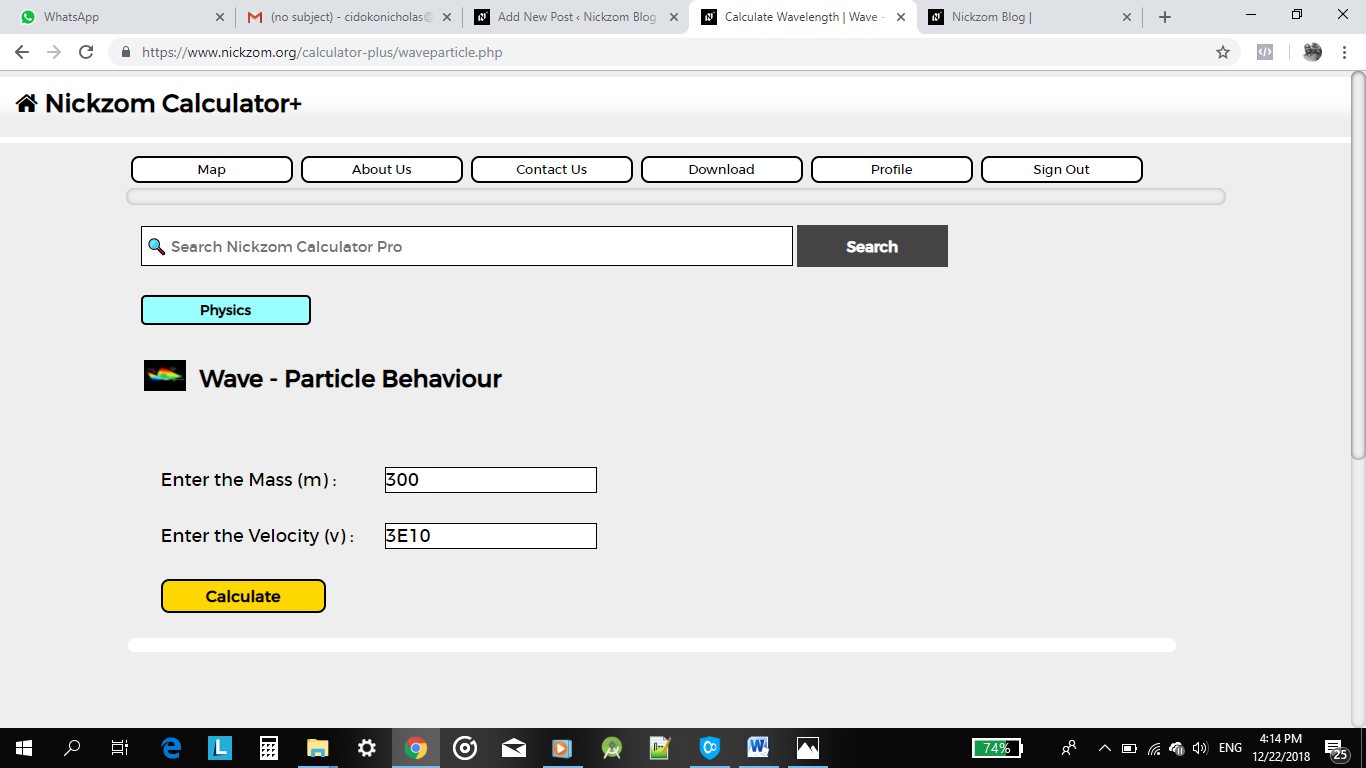The image depicts a detailed screenshot of a desktop application. In the top left corner of the screen, several browser tabs are open. The first tab is labeled "WhatsApp," indicating it might be the desktop app for WhatsApp. Adjacent to it is a tab for "Google Mail," which shows an email with no subject and the account user displayed as CitoCoNicholas, partially cut off.

Further to the right, another tab provides an option to "Add New Post for Nixom Blog." Following this, there is a tab titled "Calculate Wavelength / Wave," which is currently active, and another tab also labeled "Nixom Blog."

In the active tab, the URL displayed in the search bar reads "https://www.nickzom.org/calculator-plus/waveparticle.php," indicating the user is on the Nixom Calculator Plus site. Nixom, spelled N-I-C-K-Z-O-M, appears to be a key part of the application.

Below the tabs, the Nixom Calculator Plus application interface is visible. The upper section of the interface shows six pale rectangular buttons with black margins, labeled: "Map," "About Us," "Contact Us," "Download," "Profile," and "Sign Out."

A large search bar with a magnifying glass icon is situated beneath these buttons, containing the text "Search Nixom Calculator Pro." A black rectangular button labeled "Search" is placed to the right of this bar.

Further down, a light blue button marked "Physics" is situated prominently. Below, in bold text, it reads "Wave - Particle Behavior." The interface includes fields for entering mass and velocity, suggesting inputs for a physics calculation. A pale yellow button labeled "Calculate" is available at the bottom of these input fields.

The overall layout and labels indicate that the screenshot is from a physics-based calculator application, specifically aimed at calculating wave and particle behaviors.